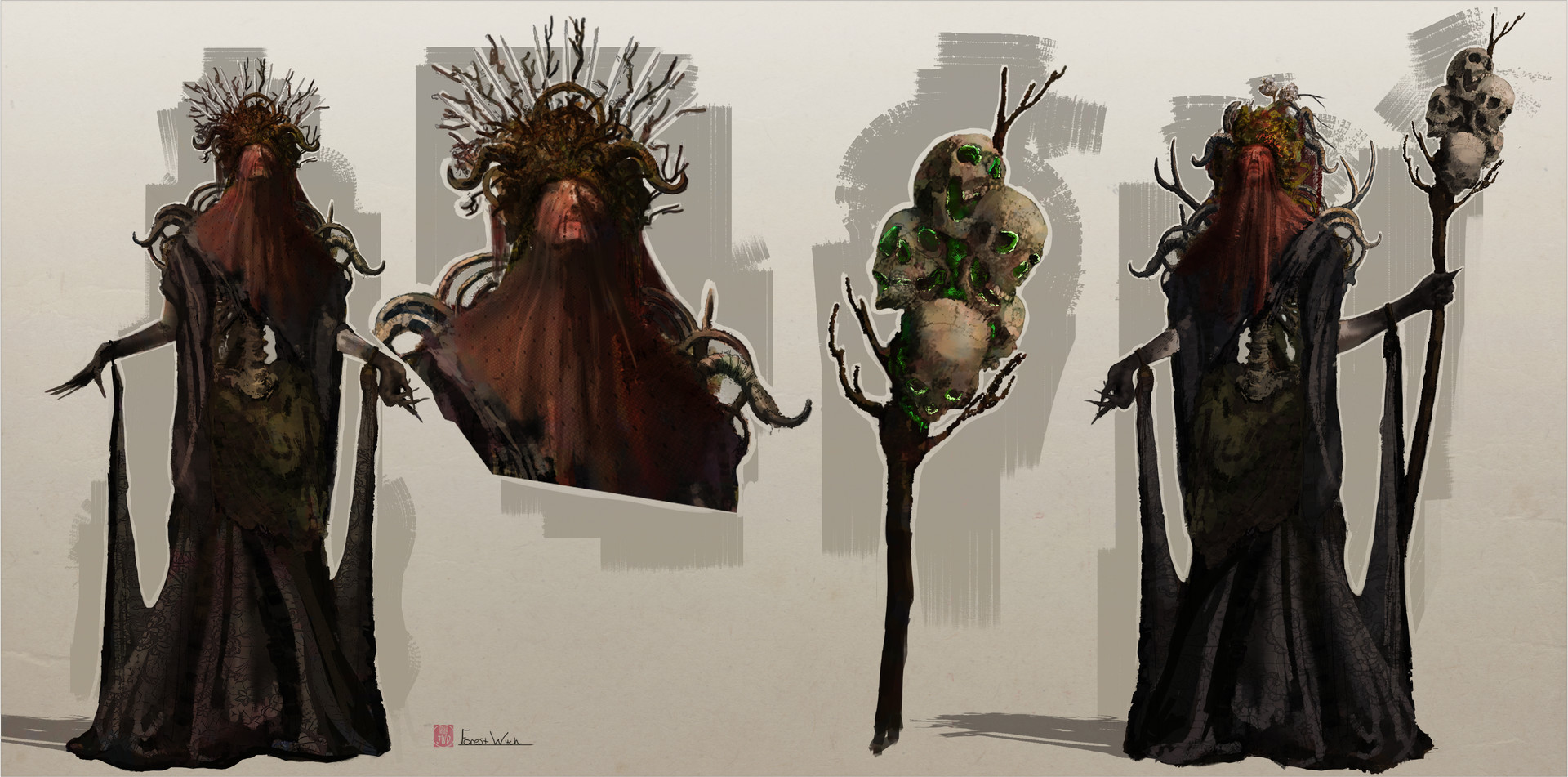The image is an intricate and surreal piece of art, composed in a panoramic dimension with multiple portrayals of an enigmatic, shaman-like figure. The background appears as simple white paper, against which the primary figure is set against a silver-gray backdrop. This main figure, reminiscent of religious or skeletal imagery, is veiled with a brown covering that partially reveals their nose and mouth. They wear a black, tattered long dress, holding its tails over their wrists, revealing spindly hands and fingers. The figure's head is adorned with a peculiar crown, seemingly composed of snakes, twigs, and horns, resembling but differing from a traditional crown of thorns. To the left, there is a detailed, zoomed-in shot of the veiled face and crown. To the right, another depiction shows the figure gazing to the left, holding an eerie branch adorned with five skulls that have glowing green eyes. The composition suggests a multi-faceted, otherworldly entity, part shaman, part skeletal apparition, wielding power and mystery through its haunting and detailed presentation.